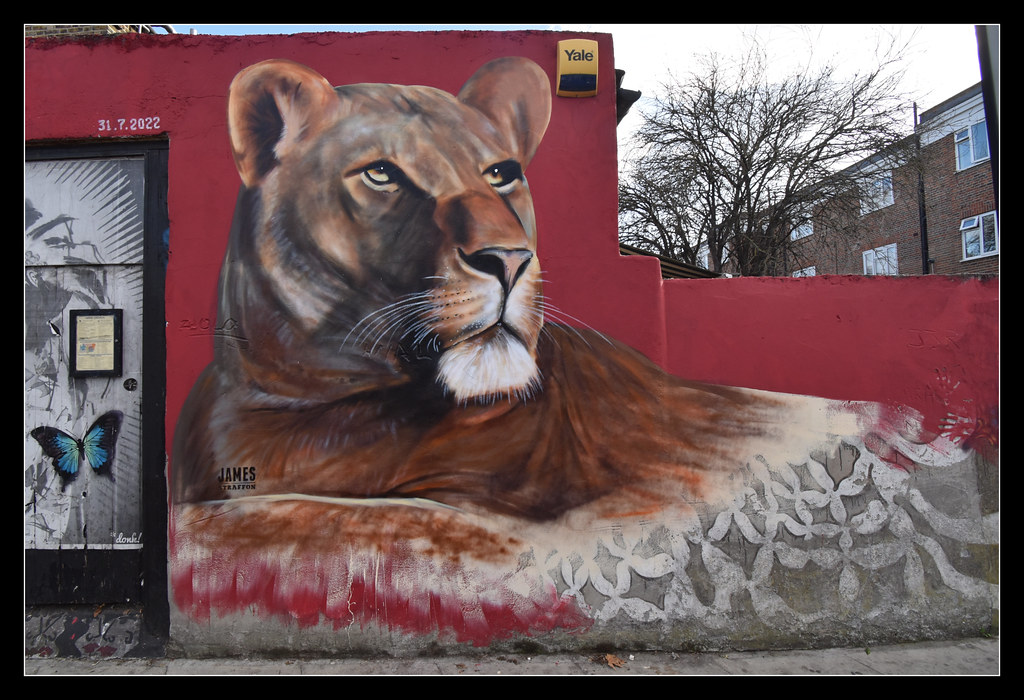The image presents a color photograph of a striking outdoor wall mural on a building. The mural features a highly realistic portrayal of a female lion, captured from the top of her ears to just below her shoulders. This lioness, depicted in a three-quarters angle, has a beige short fur coat with a brown muzzle and white fur under her chin, highlighting the detailed brush strokes that enhance the lifelike texture. The lion appears to be staring slightly to the right side of the image. Below her neck and shoulders, the painting transitions into an abstract form, resembling a white blanket with a lacy bottom, intermixed with shades of brown and red. The mural is set against a dark red wall background.

Adjacent to the mural, on the left, there is an accompanying image featuring a blue and black butterfly over a gray and white background resembling a map. Above this image is a black marquee sign. The composition also features the upper section of a mostly brick apartment building in the background, towering over the mural, with a leafless tree indicating a winter scene. The photograph is taken from a sidewalk perspective, capturing the building's side, which is single-story on the right and two-story on the left. The mural includes text elements: a little sign in black and yellow in the top corner of the wall reading "yell," a door with additional signage beneath, and the date "31.7.22" above the door, suggesting the mural's completion date. There's a name on the chest of the lion in black letters, reading "James," though the remaining text is too small to decipher. The overall style of the mural reflects photographic representationalism and realism.